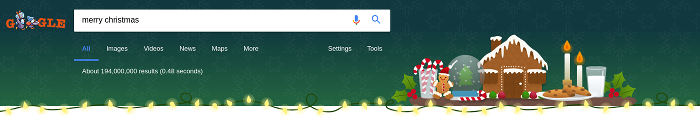The image features the top section of a web page with a Google search. It is a long, narrow, greenish rectangle, starting from a deep hunter green at the top and gradually transitioning to a lighter shade of green towards the bottom. The green hue resembles that of pine trees, evoking a Christmas ambiance.

In the top right-hand corner of the rectangle, the word "Google" is displayed in all capital letters, uniquely rendered entirely in red, deviating from its usual multi-colored format. Cleverly, the two 'O's in "Google" are replaced with illustrations of Christmas packages, reinforcing the festive theme. A search bar beneath the logo contains the typed phrase "Merry Christmas."

Below the search bar, the word "All" is highlighted in blue with an accompanying blue line, indicating it is the selected category. The search results indicate approximately 1,194,000,000 results, however, only the interface elements are visible in the picture, not the actual results. Options such as "Images," "Videos," "News," "Maps," "More," along with "Settings" and "Tools" are clearly visible.

To the right of these options, a colorful, Christmassy image is displayed, featuring a gingerbread house adorned with cookies, candy canes, a gingerbread man, and a snow globe, enhancing the overall holiday spirit of the scene.